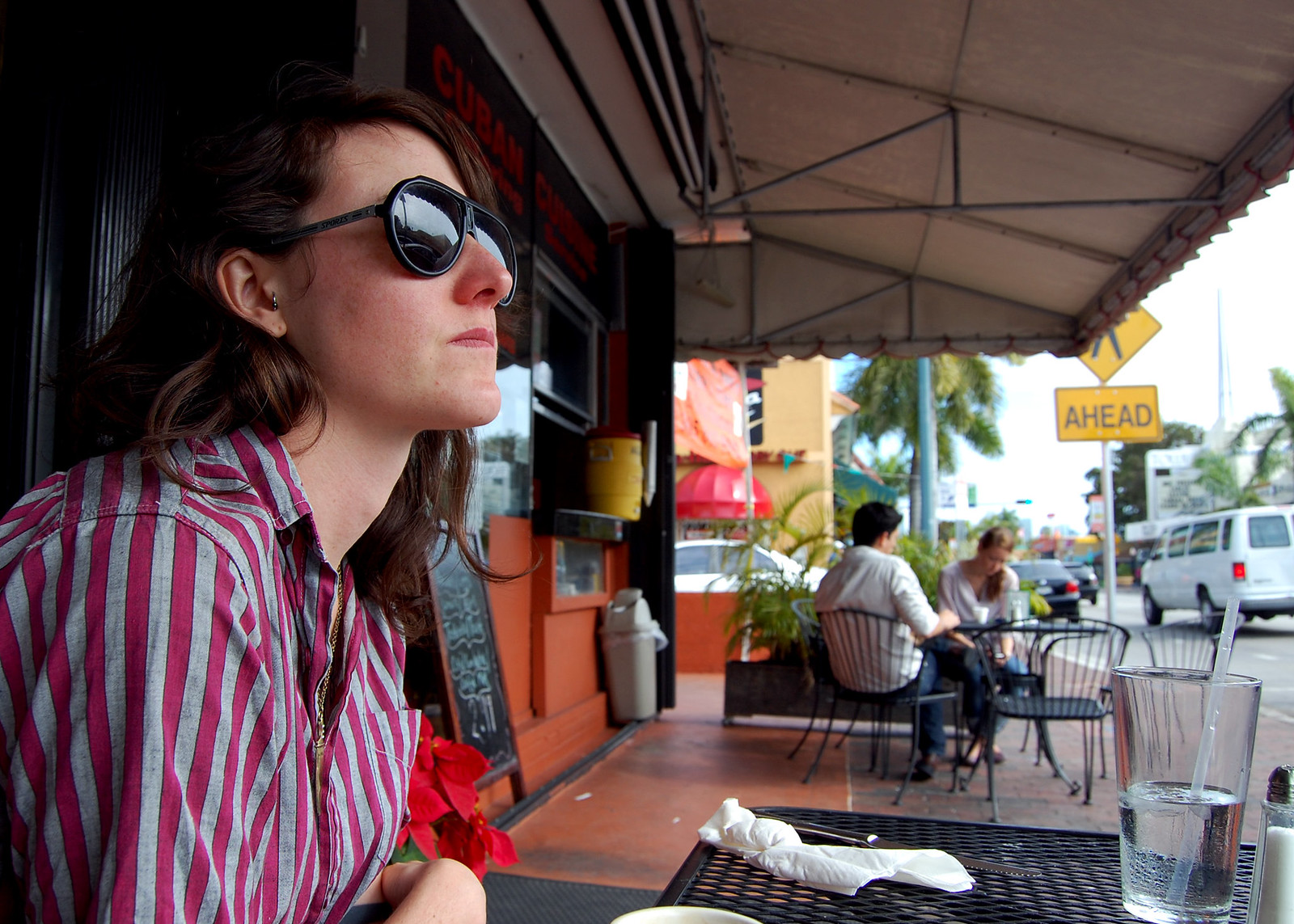This photo captures an outdoor scene at a restaurant or coffee shop patio during the daytime. The primary subject is a young Caucasian woman with tousled, shoulder-length brown hair, wearing black sunglasses and a purple and gray vertical striped button-down shirt. She is seated at a black metal table with a grid pattern, which holds a crumpled white napkin and a half-full glass of water with a straw. The woman is facing to the right, with her back towards the restaurant on the left. Her chin is tilted upward slightly, and she appears to be resting her hand on the table.

In the distance, another outdoor table seating a Caucasian man and woman can be seen. The man has dark hair, while the woman has either dark blonde or light brown hair, and they are also seated at black metal furniture. The restaurant, painted red, provides the backdrop for these tables.

To the right side of the image, a street with palm trees and cars, including a visible white van, extends into the distance. A yellow "AHEAD" crossing sign is visible near the road. The entire patio area is shaded by an awning, providing a bit of shelter to the people seated beneath it.